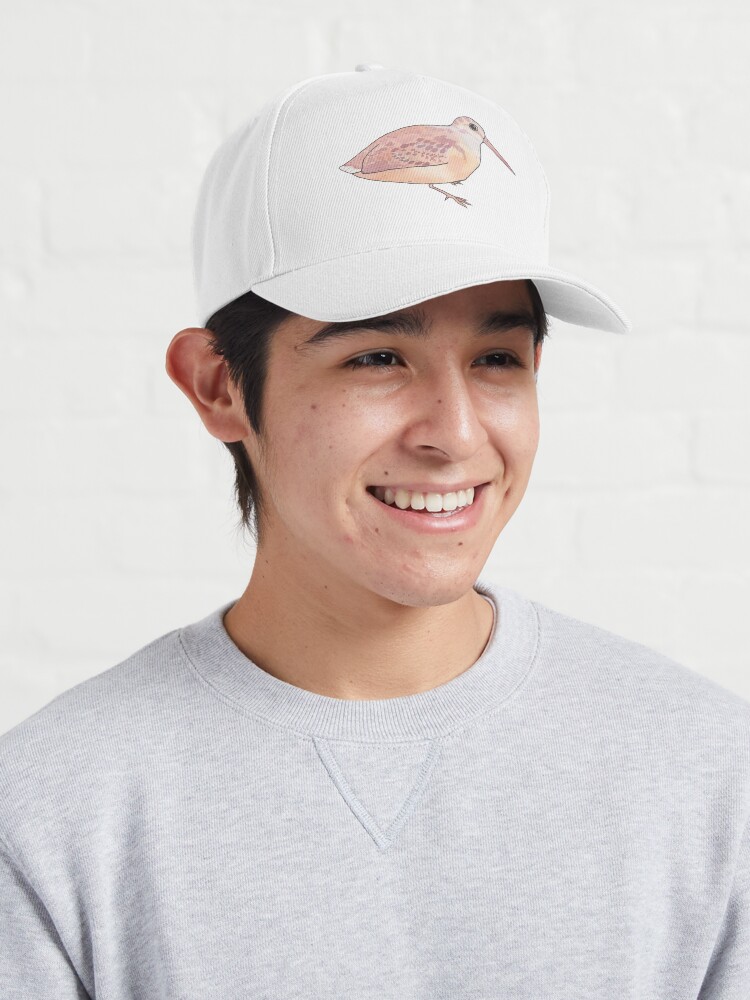This is a close-up portrait of a young male, likely in his mid-teens (around 16 or 17 years old), with short dark hair and dark eyebrows. His hair peeks out just below a white baseball cap that features a small, detailed bird design in the center. The bird is characterized by a long, pointy beak, a black eye, an orangey-white head, a white neck, an orangey belly, and pinkish wings. The cap is textured and fits snugly on his head. 

The young man is sporting a light, heather gray crew neck sweatshirt that is slightly loose-fitting, with a noticeable triangle detail beneath the neckline. He has a pleasant smile that reveals his white teeth. His face is adorned with a few freckles, pimples, and prominent dimples that are visible due to his cheerful expression. He is slightly turned to the left, enabling a clear view of his right ear, which appears relatively large. The background of the image is plain white, overall giving the portrait a clean and simple look.